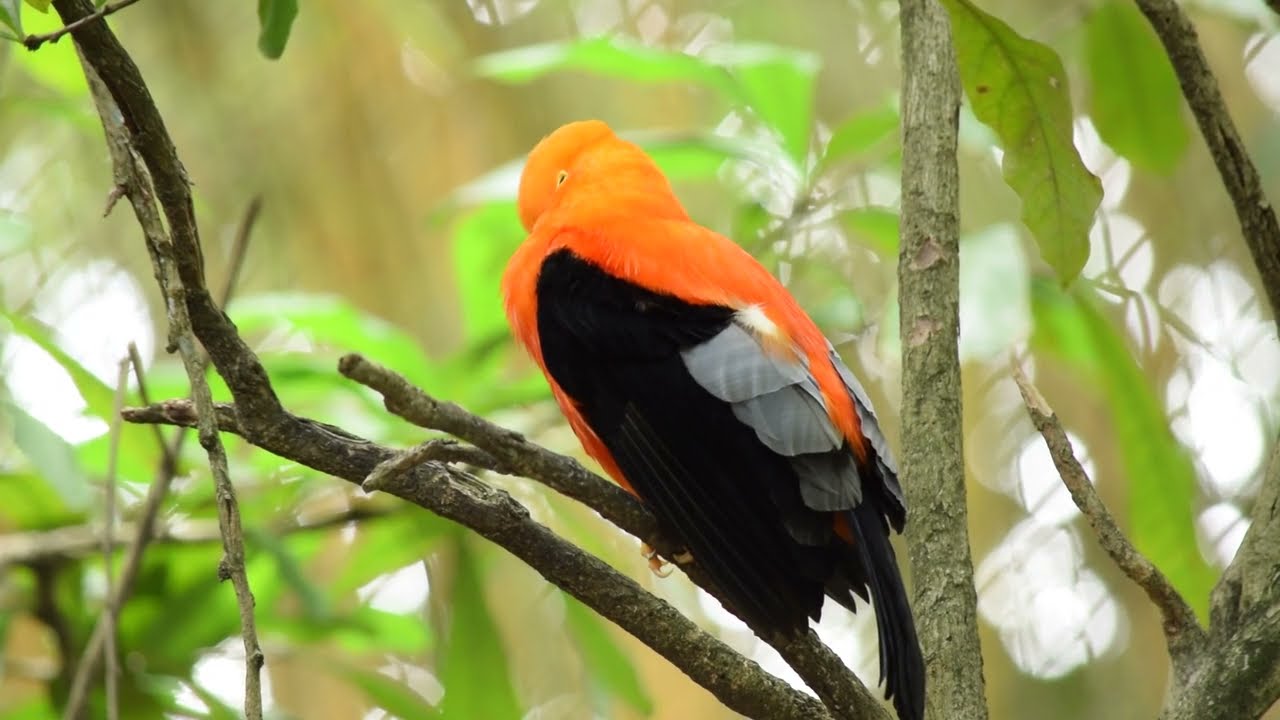In this vibrant outdoor photograph taken during the daytime, a striking tropical bird stands out as the central focus, perched gracefully on a tree branch. Its plumage is an eye-catching combination of vivid colors: the head, neck, and shoulders are a deep orangish-red, while the breast showcases bright orange hues. The bird’s wings and tail are predominantly black, speckled with white and grey highlights, giving it a unique and beautiful palette. Its eyes are closed, indicating it is peacefully sleeping with its beak nestled into its feathers. The detailed backdrop showcases lush green foliage, with hints of yellow leaves, suggesting a dense, tropical environment, possibly akin to a nature preserve or wilderness setting. The background trees appear slightly blurred, further drawing attention to the exquisite bird nestled among the greenery.